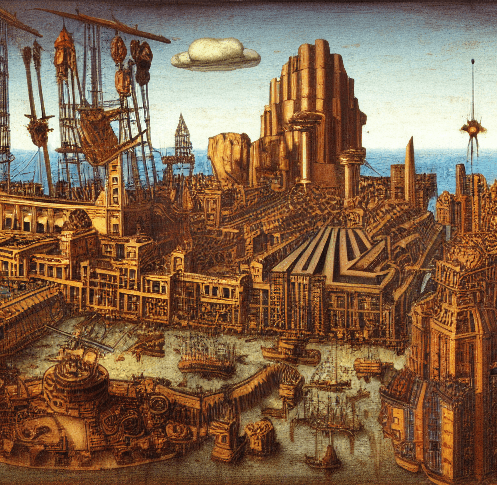This image is a detailed painting of an ancient, bronze-age style city featuring a grand, multi-story central structure resembling a castle or industrial tower surrounded by lower rooftops and various steeples. The city, possibly retro-futuristic or even fantasy, is perched by a body of water with visible ships, suggesting it's a bustling port. The water near the port is greenish, while the water in the distance is vibrantly blue. The gray-blue sky at the horizon fades into white, adorned with a single puffy cloud near the iconic segmented cylindrical tower in the background. Additional elements include a small courtyard with wooden structures, an intricate maze-like area, and an assortment of mysterious buildings giving the entire scene an air of complexity and rich architectural diversity.